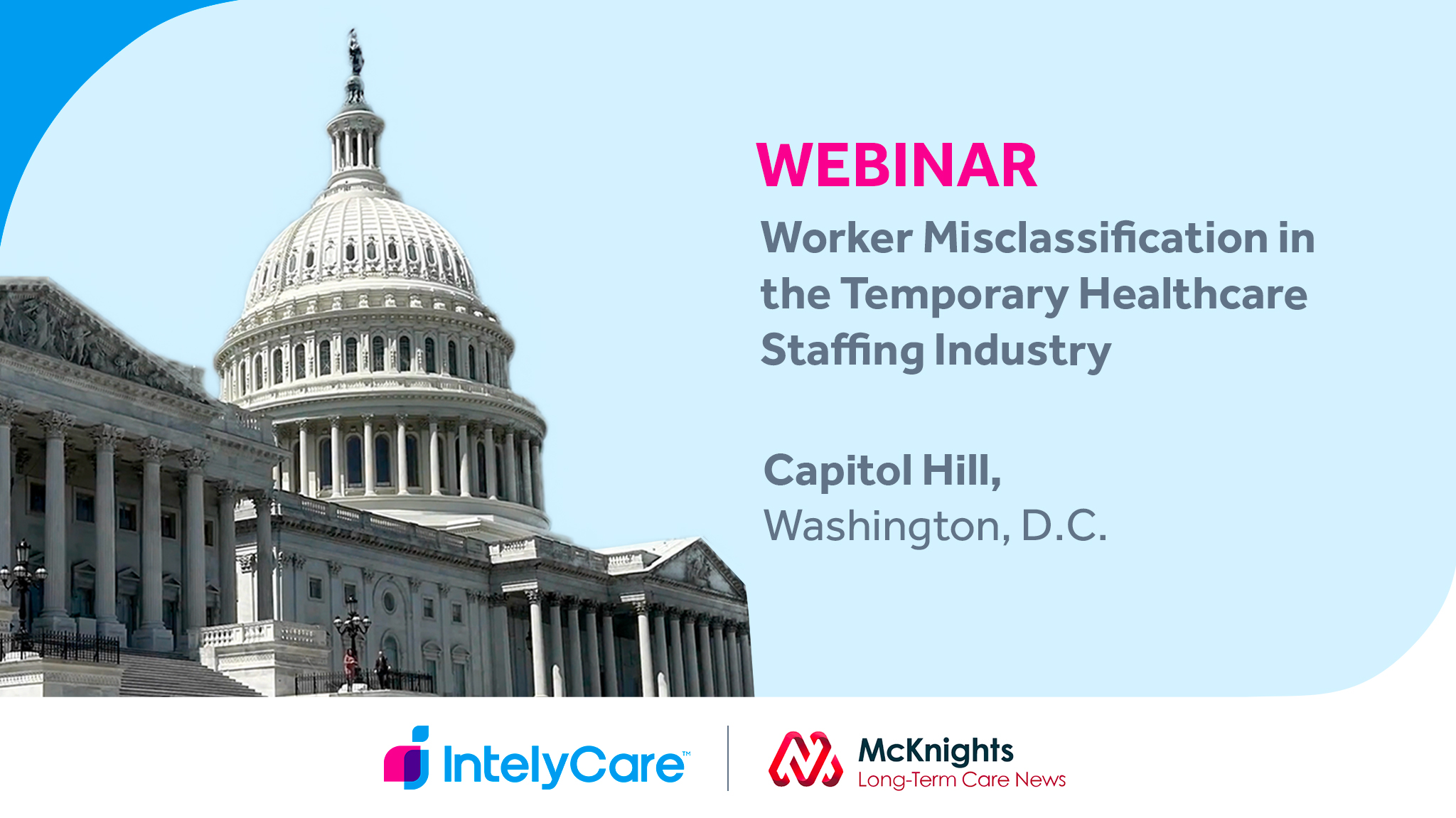This advertisement slide for a webinar features a light blue background with the iconic U.S. Capitol building prominently displayed on the left side, showcasing its ornate architecture, carvings, and pillars, along with visible lights and the balcony. The headline "WEBINAR" is in bright hot pink all caps, followed by the topic "Worker Misclassification in the Temporary Healthcare Staffing Industry" in gray, left-aligned font. The location is specified as "Capitol Hill, Washington, D.C." Below the text, the logos of IntelliCare, with their blue and pink design, and McKnight's Long-Term Care News, with red and black lettering, are separated by a vertical line and positioned outside the main color block. The advertisement is characterized by its square corners on three sides, with the bottom right-hand corner distinctly rounded.